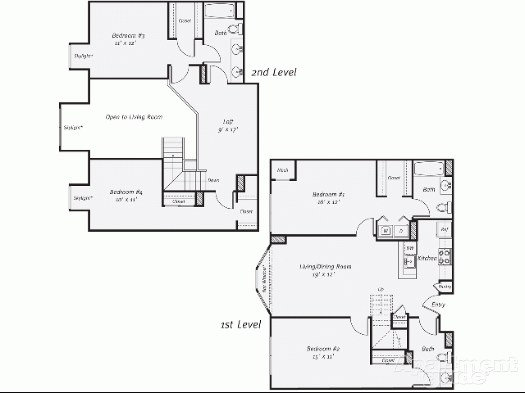This blueprint image depicts the architectural plan of a house, displayed on a white background with predominantly black outlines and some elements shaded in gray. Despite the image being blurry and pixelated, certain details are discernible.

In the lower right corner, the blueprint is labeled "First Level" and shows a rectangular outline of the house. Above this label, there appears to be a bay window, though the details are unclear due to the image quality. The text "First Level" is positioned on the left side of this outline. Moving rightward within the plan, there is an entryway that opens into a combined living and dining room, which measures approximately 19 feet by 12 feet. Directly below this living area, there is a space that could either be a bathroom or bedroom, approximately 25 feet by 12 feet. At the very top of the first level, there is another room labeled "Bedroom 2," also measuring 25 feet by 12 feet. There are various features extending from this bedroom, but the pixelation makes them illegible.

On the upper left side of the blueprint, details of the "Second Level" are noted. The text indicating "Second Level" appears to be to the right of this section. At the top left of the second level, there is a space labeled "Bedroom," measuring roughly 22 feet by 22 feet. Directly below this bedroom, a note reads "Open to Living Room." To the right of this space, there is an area possibly designated as a "Loft." Below the loft area, there might be another label for "Bedroom 4," though this is not entirely clear due to the pixelation.

Overall, the blueprint provides a general layout of both the first and second levels of the house, featuring several rooms with specified dimensions and a mix of open and labeled areas, despite the struggling legibility of specific sections.